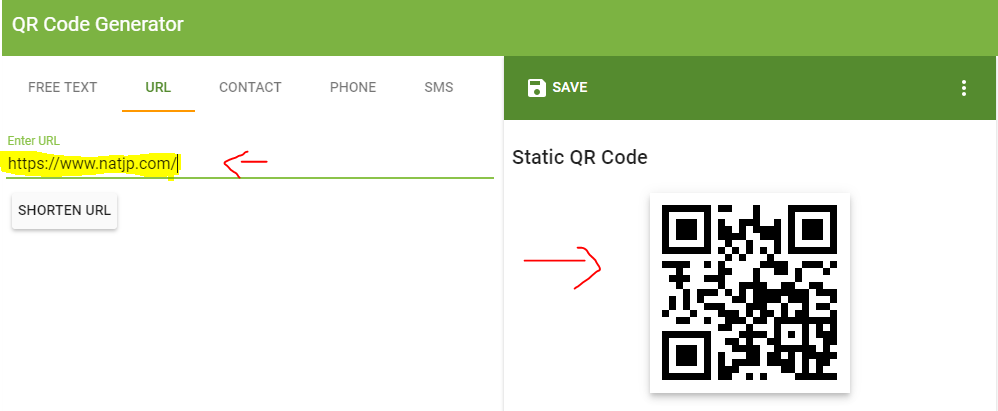The image appears to be a screenshot of a computer screen displaying a QR code generator interface. At the very top, the interface features a long light green band, with the text "QR Code Generator" situated in the left corner. Below this band, there are five selectable options, listed as follows: "Free Text," "URL," "Contact," "Phone," and "SMS." The "URL" option is prominently underlined in red.

Beneath the selection menu, there is a text field labeled "Enter URL," where the user has entered the URL: "https://www.natjp.com/". A hand-drawn red arrow points to this URL entry field. Below the URL entry, there is a button labeled "Shorten URL."

On the right side of the screen, a dark green vertical band appears, displaying the word "Save" with an ellipsis (three dots) stacked vertically beside it. Additionally, it mentions "Static QR Code." Adjacent to this text is a square containing the graphical representation of a QR code, featuring intricate black patterns and three prominent black squares, located at the upper left, upper right, and bottom left corners of the code. A hand-drawn red arrow points to this QR code, emphasizing its presence.